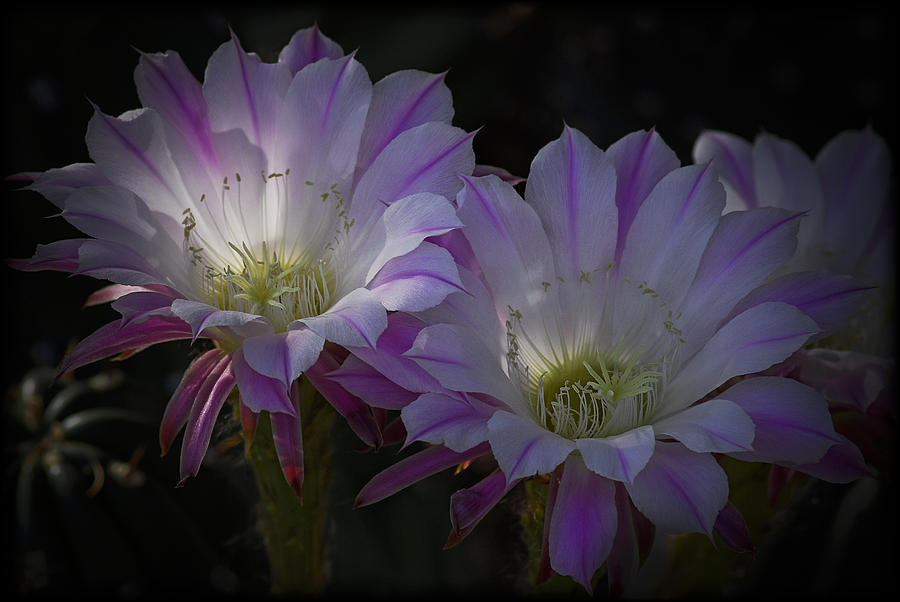This image is a close-up photograph of two prominent blooming flowers, positioned side by side, each with their centers slightly angled upwards towards the viewer. The flowers are primarily white but feature striking pink or purple veins running down the petals, and they exude an ethereal glow, suggesting the light may be coming from behind or the side, highlighting their detailed structure against an entirely black background. The flowers boast numerous petals, each one gracefully open, and the centers are filled with delicate, grass-like white stems that have green tips, alongside many yellow stamens. There's also a faint presence of another flower to the right in the background, slightly out of focus. The black backdrop and the emphasis on the incandescent appearance of the flowers suggest a possible use of filters to enhance the contrast, making the blossoms stand out luminously.